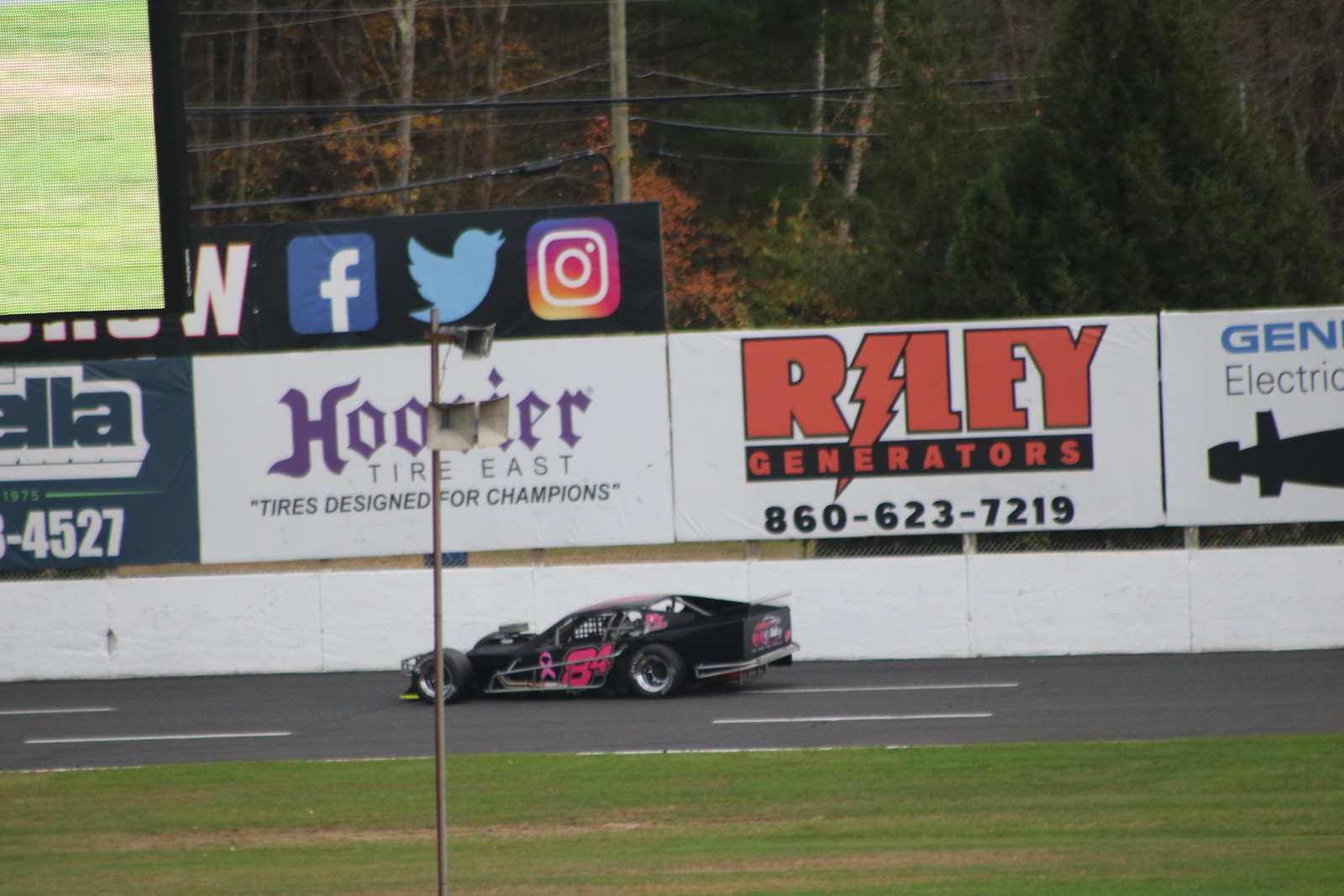The image captures a dynamic scene of a black race car speeding around a racetrack, moving from right to left. The car features notable pink graphics, including a number that looks like 50 something, comprised of the numbers 8 and 4, and a pink ribbon symbolizing breast cancer awareness. The side of the car is adorned with various numbers and advertisements. In the foreground, the green grass of the infield is visible along with the black track lined with white stripes. A pole with a speaker is seen at the bottom left of the image. Beyond the car, the white track border is visible, above which there is a large fence bearing multiple advertisements. The large fence displays signs for Hoosier Tire East, "tires designed for champions," Riley Generators with the contact number 860-623-7219, and social media emblems for Facebook, Twitter, and Instagram. The background stretches to a wooded area filled with trees, with a patch of grassy terrain in the upper left corner of the image.